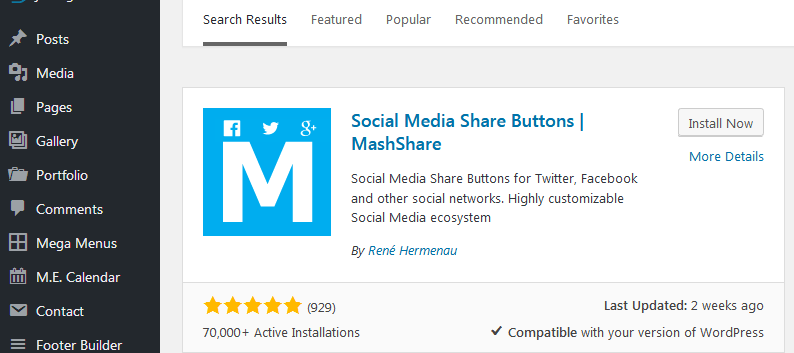The image is a horizontally rectangular partial screenshot of an application interface. On the right side, there's a vertically rectangular section with a black background displaying a vertical list of options, including "Posts," "Media," "Pages," "Gallery," "Portfolio," "Comments," "Mega Menus," "ME Calendar," "Contact," and "Footer Builder." 

The remainder of the frame features a top section with a white background. The "Search Results" option is underlined in black, indicating it is the active selection. Other options like "Featured," "Popular," "Recommended," and "Favorites" are listed next to it.

Beneath these options on the white background, there are social media share buttons labeled "Match" and "Share." To the left of these buttons, there is a blue box with a large "M" in it, accompanied by icons for Facebook, Twitter, and Google Plus above the "M."

A description below mentions "Social media share buttons for Twitter, Facebook, and other social networks. Highly customizable social media ecosystem."